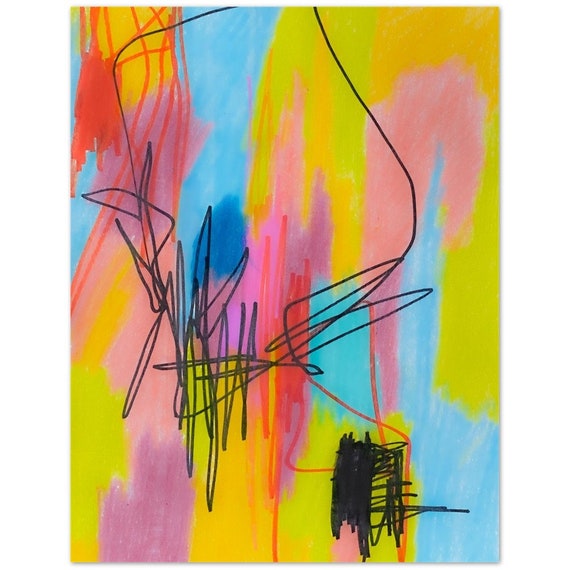This piece of abstract art features an array of vibrant colors layered in a polychromatic pattern with predominantly vertical strokes. The background showcases a diverse palette that includes shades of yellow, orange, peach, blue, magenta, dark red, neon pink, lime green, and various tones of purple. These hues are applied in irregular, overlapping splotches, creating a dynamic and intricate pattern. Superimposed on this colorful backdrop is a chaotic overlay of black sharpie scribbles, giving the appearance of disruptive, jagged, zigzag lines. Additionally, there are noticeable squiggles in red and possibly orange. The overall effect is non-representational, presenting a collage of bright, cheerful colors with random black markings. In the bottom right corner, a conspicuous black box is drawn and filled in, adding to the sense of disorder and spontaneity in the composition.